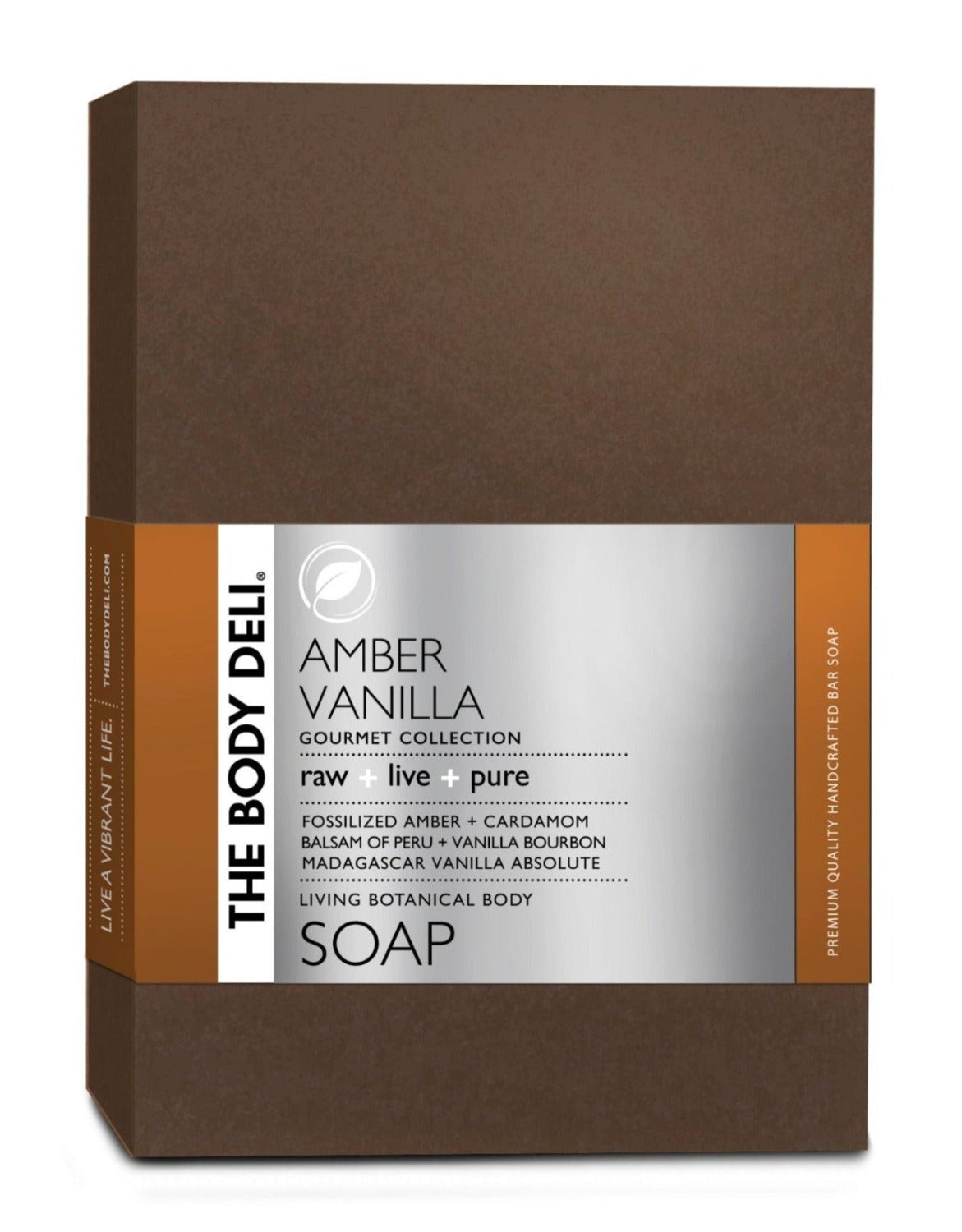This image depicts a high-end, handcrafted bar of soap standing on end. The soap has very square corners, suggesting it may be handmade and cut into blocks. It features a dark brown color and is wrapped in a sophisticated cardboard label. The label, predominantly gray, includes areas of dark muted orange on either side, almost like the spine of a book. The central portion of the label reads "The Body Deli Amber Vanilla Gourmet Collection" and highlights the ingredients: fossilized amber, cardamom, Balsam of Peru, vanilla bourbon, and Madagascar vanilla absolute. Descriptive terms such as "raw," "live," and "pure" emphasize the natural and premium quality of the soap. The side of the label boasts "Living Botanical Body Soap" and "Premium Quality Handcrafted Bar Soap." The texture and presentation suggest an exclusive and luxurious product.